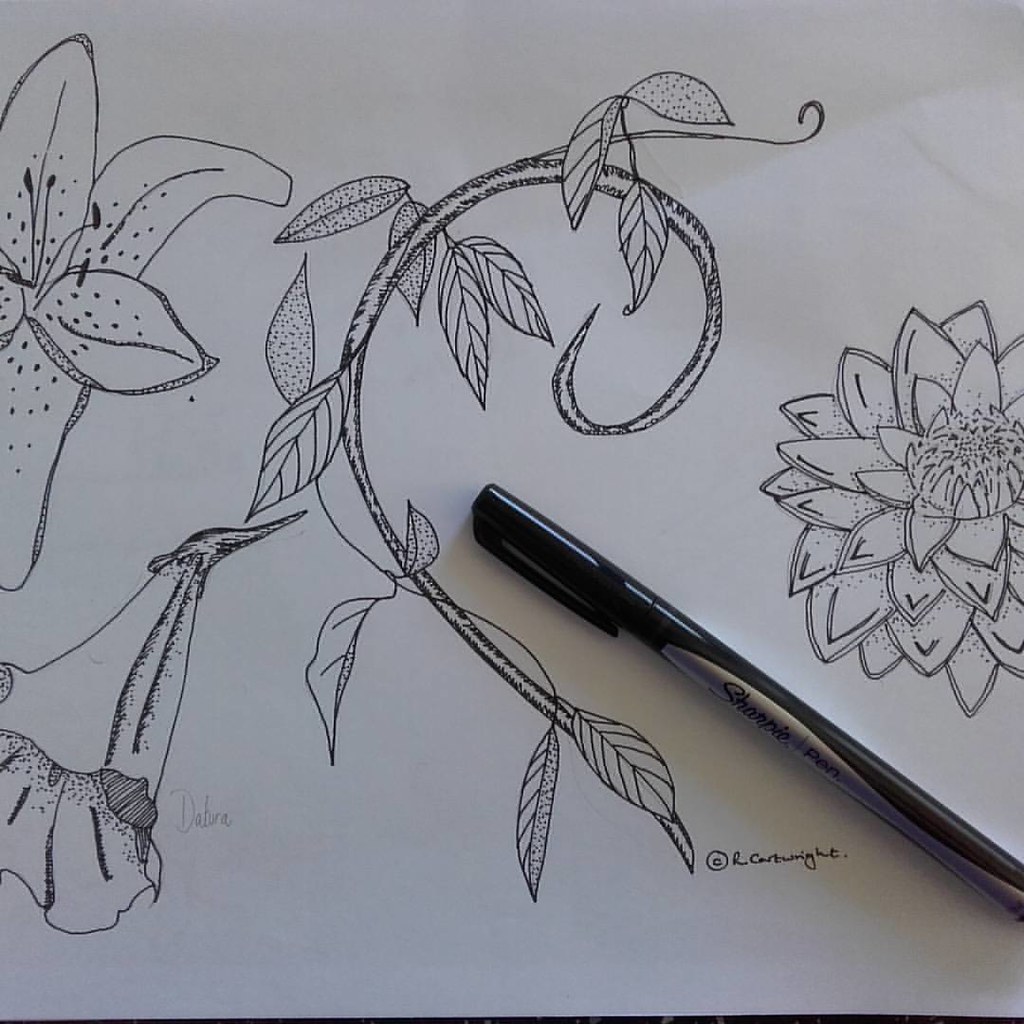This image features an intricate pen and ink drawing rendered entirely in black ink on a white paper background. The botanical design prominently showcases flowers, vines, and leaves. On the left side of the drawing, a large lily stands out with detailed petals and stamens. The center of the composition is filled with winding vines adorned with delicate leaves, some of which have smaller vine patterns within them. To the right, there is a beautifully detailed dahlia with layers of tiny, precise petals. Resting atop the drawing is a black Sharpie pen, identifiable by the silver branding on its body. The artwork is rich in detail, with clear, meticulous lines that emphasize the textures of the petals and leaves. No human figures or additional text are present within the artwork, but it is signed by the artist, adding a personal touch to this botanical masterpiece.